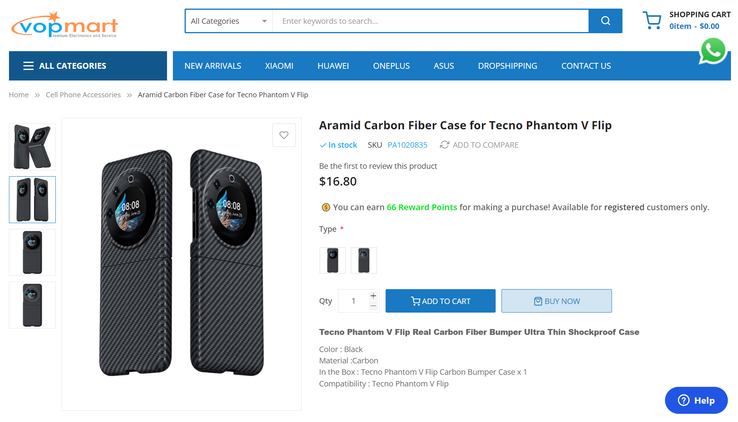A website screenshot featuring VOP Mart is displayed. The background is predominantly white, complemented by a vibrant header. At the top left, the website name "VOP Mart" is prominently presented in a mixture of blue for "VOP" and orange for "MART," accompanied by a decorative star above it. Centrally positioned is a lone search box, facilitating easy navigation. To the right, an icon of a shopping cart is visible, currently indicating an empty cart with a value of 0.00.

Below this header are two distinct horizontal sections. The first section is a dark blue bar that includes a dropdown menu titled "All Categories." Adjacent to this is a lighter blue navigation menu, offering clickable links to various sections such as "New Arrivals," "XIAOMI," "HUA" or "HUI," "OnePlus," "Asus," "Drop Shipping," and "Contact Us."

Beneath these menus, the main content area showcases a product with a white background. On the left side, multiple images of a phone are displayed, including detailed shots from different angles. Adjacent to these images, the product's main photo is highlighted. On the right, product details are outlined with a heading that reads "Airmint Carbon Fiber Case for Techno Phantom V Flip." It is stated that the item is in stock, and the pricing information is provided. Below this, there are interactive buttons for "Add to Cart" and "Buy Now." Additional information about the phone can be accessed via a blue help button.